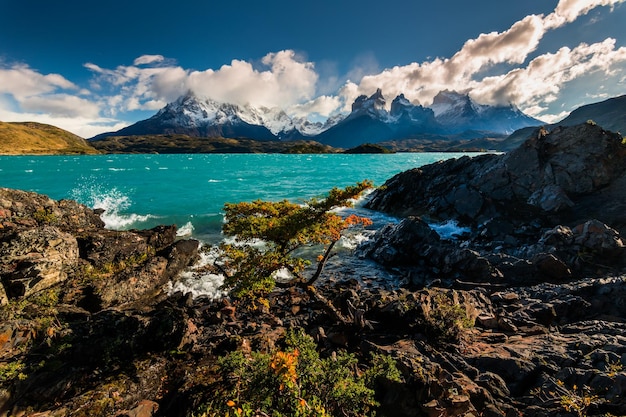A breathtaking mountainous landscape unfolds beneath a striking blue sky dotted with clouds, which cascade over majestic, snow-capped mountain ranges in the background. Centered within this serene scene is a pristine, aqua-turquoise lake, surrounded by rocky banks and green vegetation. The foreground is characterized by an array of grayish-brown rocks and patches of greenery, with a notable tree branch extending over the water on the right side, where waves gently splash against the stones. This vibrant portrait captures the essence of natural beauty, evoking a sense of tranquility and untouched wilderness.